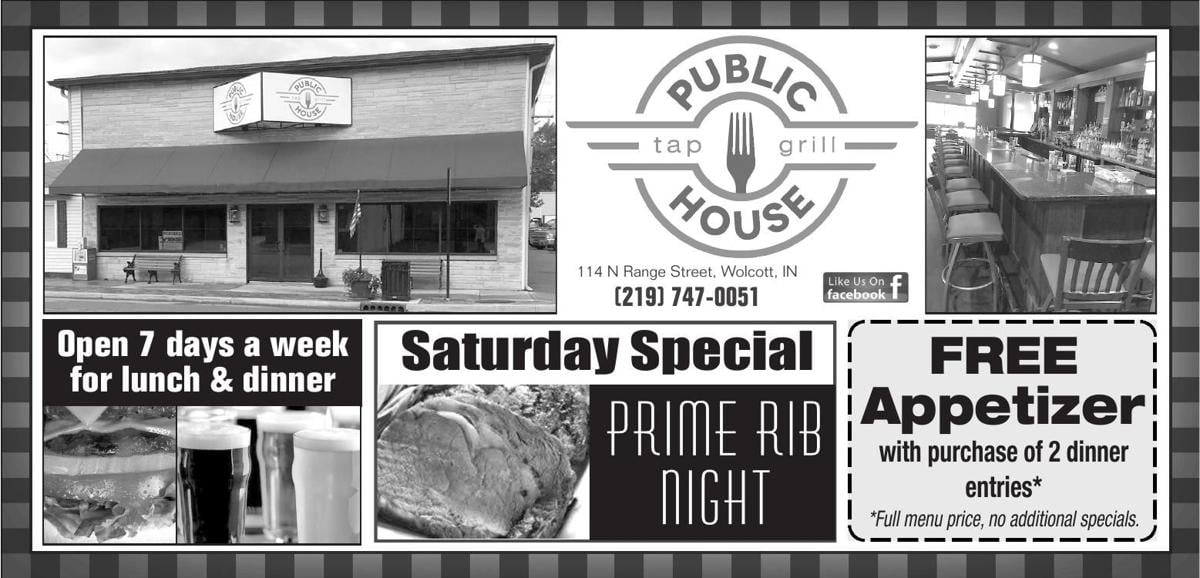This black and white advertisement for "Public House Tap Grill" in Walcott, Indiana, prominently displays various details about the restaurant. On the left side, there's an image of the storefront, featuring a black or dark gray awning, two benches, an American flag, and a garbage can. There is signage visible from both directions of the street, stating "Public House Tap Grill" in a circular design with a fork in the center. Adjacent to this is the restaurant's logo along with its address, 114 North Range Street, and phone number, 219-747-0051.

The advertisement also shows the interior of the restaurant, highlighting a long wooden bar with numerous bar stools. An overlay text informs that the establishment is "Open seven days a week for lunch and dinner." In the middle of the ad, there is a section that focuses on their offerings, mentioning a Saturday special for prime rib night accompanied by a picture of the dish. At the bottom right corner, a coupon offers a free appetizer with the purchase of two dinner entrees at the full menu price, specifically noting that no additional specials can be combined. The advertisement also includes images of food and glasses of beer to entice potential customers.